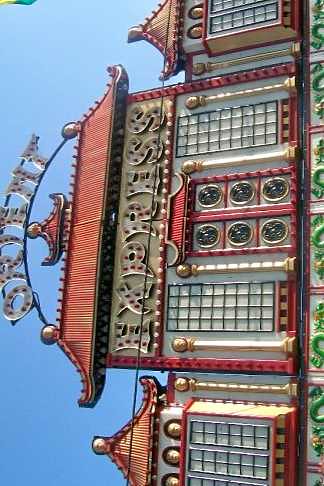This photograph captures the intricate façade of a Chinese restaurant, featuring a sign designed to resemble traditional pagoda-style architecture. The sign structure is adorned with characteristic red-tiled roofs with upward-curving eaves, evoking the classic aesthetic of Chinese pagodas. Below these roofs, the restaurant's main entrance is highlighted by an elaborate, centrally placed door, crowned with another pagoda-style roof and flanked by two ornamental poles. The door itself is composed of silver panels, each bearing three rounded lights.

At the pinnacle of the sign, an archway displays the word "Orient" in illuminated lettering. Just beneath the main red roof section, the word "Express" is similarly outlined with light bulbs, ready to shine. The vibrant composition of the scene stands out prominently against a bright blue sky, with the primary colors of the façade being whites, golds, and reds, making for a visually striking and culturally evocative image.